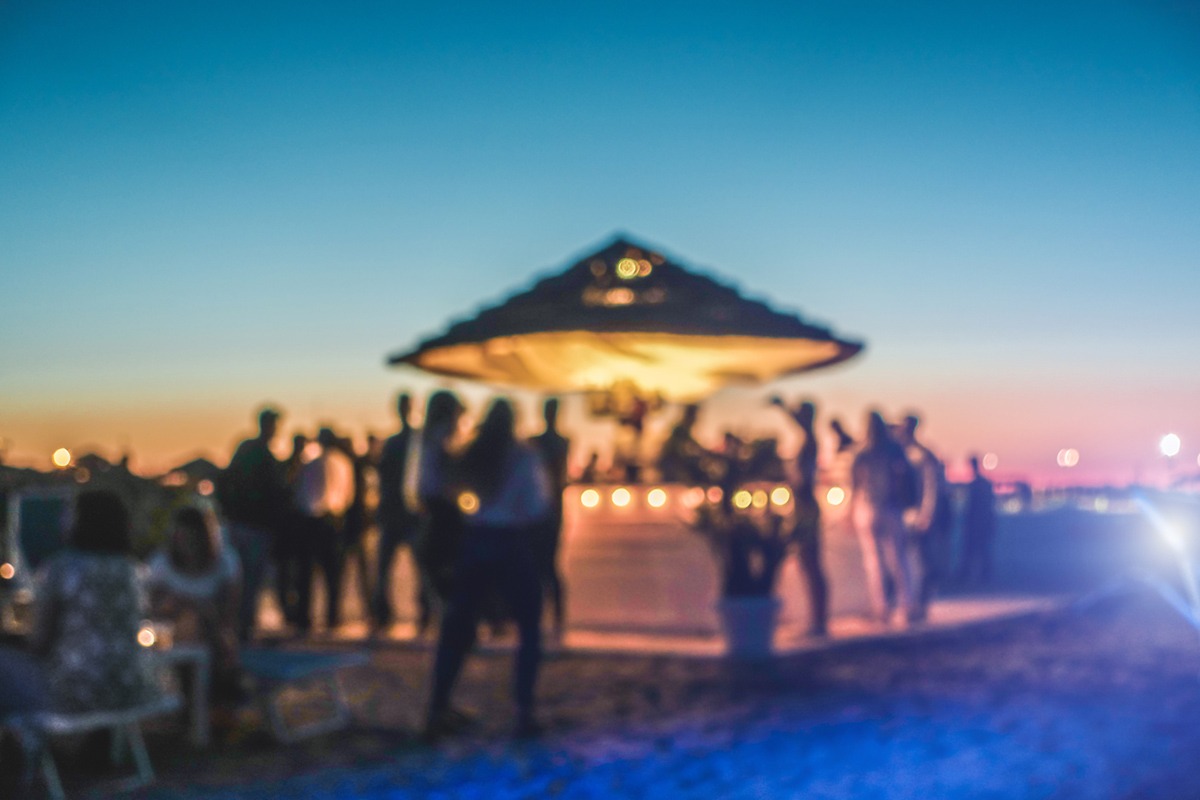This horizontally aligned, out-of-focus photograph captures a bustling beach scene during the early evening. At the center of the image, there's an outdoor bar or kiosk setup, situated on a wooden platform, giving off a tiki-torch vibe with a lit umbrella or gazebo overhead. The structure is adorned with globe string lights, casting a warm, yellow hue across the area. Around this bar, 20 to 30 people can be seen mingling, adding to the lively atmosphere. 

In the lower left corner of the image, a table with benches is occupied by a couple of women, possibly sitting on recliner-style beach chairs. The surrounding ground appears sandy, reinforcing the beach setting. On the right side of the photo, a bright light source washes out some of the details, illuminating the sand with a blue tinge.

The sky above transitions from a dark blue at the top to a light blue, peppered with pinkish clouds, down towards the horizon, which glows with hues of orange and yellow, indicating the photo was taken shortly after sunset. The image, though blurry, encapsulates a vibrant, outdoor beach gathering with a relaxed yet festive ambiance.